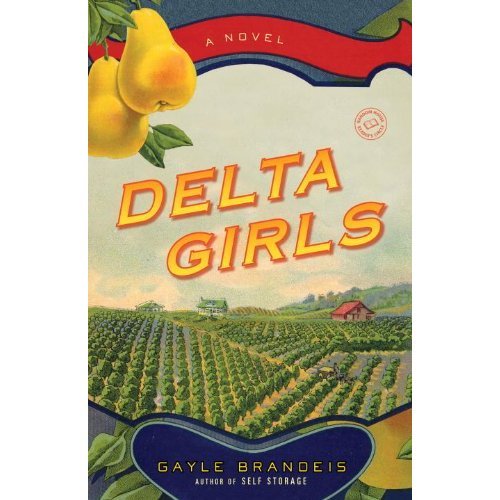The image is the cover of the book "Delta Girls" by Gail Brandeis. The title "Delta Girls" is prominently displayed in large yellow and orange capital letters at the center of the cover. A red banner in the upper portion of the cover states "A Novel" in capital letters. In the upper left corner, there are two yellow pears with a hint of orange, attached to branches with green leaves. The main background depicts an expansive field of crops, featuring rows of green shrubs typical of an orchard or farm. In the distance, there are three houses: two white ones with green roofs and one light brown house with a red roof. These houses are set against rolling hills and a sky filled with grey and white clouds. At the bottom of the cover, Gail Brandeis’ name is written in white letters, identifying her as the author of "Self Storage." Additionally, there is a red circular logo with an open book icon featured on the cover.